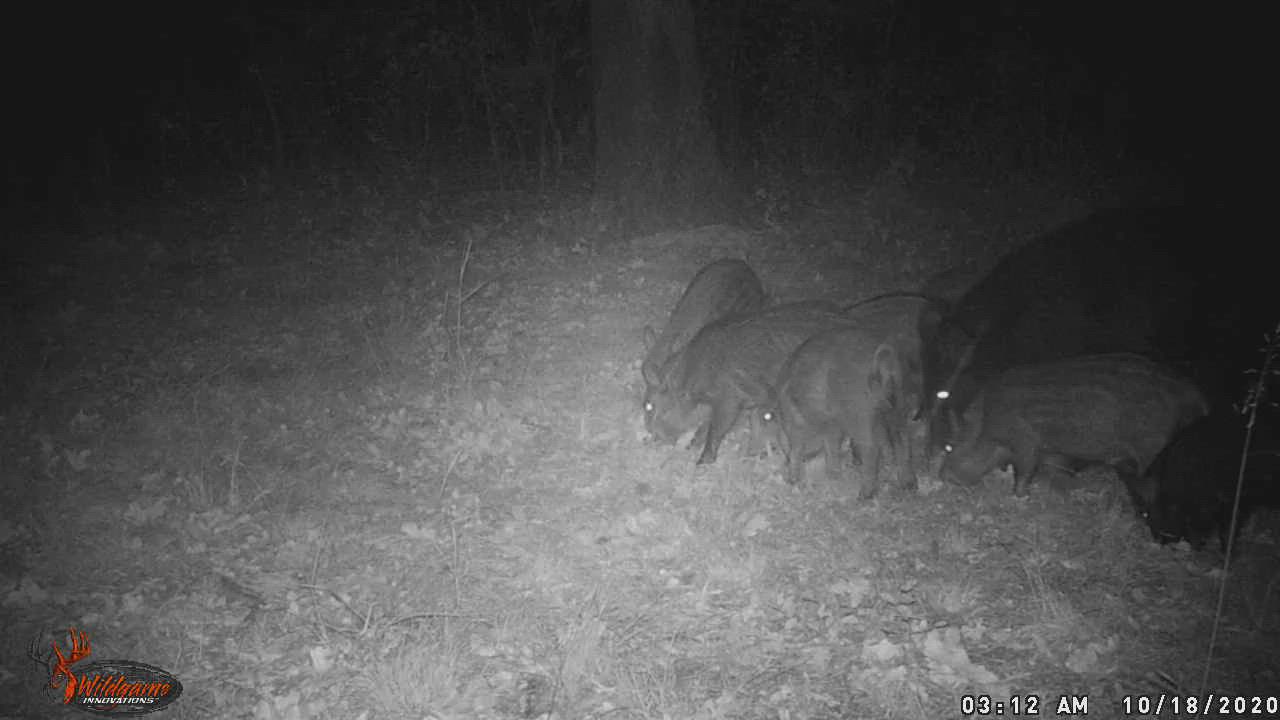This is a horizontally-oriented, black-and-white photograph taken at night using a low-quality outdoor camera, possibly a wildlife camera. The timestamp in the bottom right corner reads 3:12 AM on 10-18-2020. In the lower left corner, there is a logo with the text "Wilderness Game Interventions" - "Wilderness Game" in red and "Interventions" in white, next to a half-black, half-red deer image. The scene captures a field with grass and some trees visible in the background. Several animals, likely four or five, appear on the right side of the image extending towards the center. These animals look somewhat like pigs, although some descriptions suggest they might be bears, with one larger dark-colored figure, possibly a mother, and smaller light-colored ones, possibly cubs. Their eyes reflect brightly, indicating the camera's night vision capabilities. The image is blurry and double-exposed, adding to the difficulty in identifying the animals.